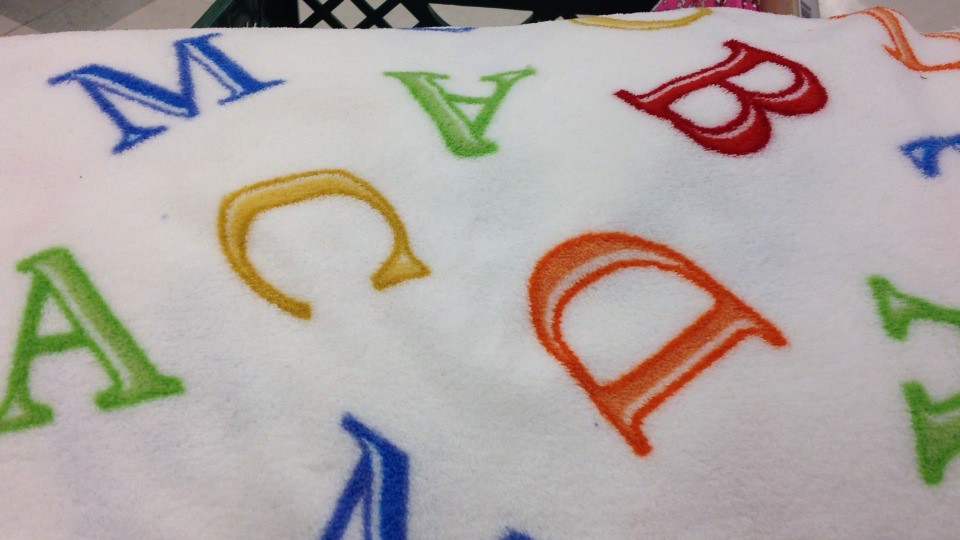The image features a detailed close-up of a white baby blanket adorned with various letters of the alphabet in different colors. Visible letters include green A's, a red B, yellow C's, orange D's, and blue M's, suggesting a playful and educational design. The letters are brightly colored: red, orange, yellow, green, and blue. The scene extends to a cozy living room setting, with the blanket draped over a chair, indicating a typical home environment. Slightly behind the blanket, there's a glimpse of a black milk crate and the floor. The photograph is vibrant yet has a slight darkish tint, adding a vintage feel to it.